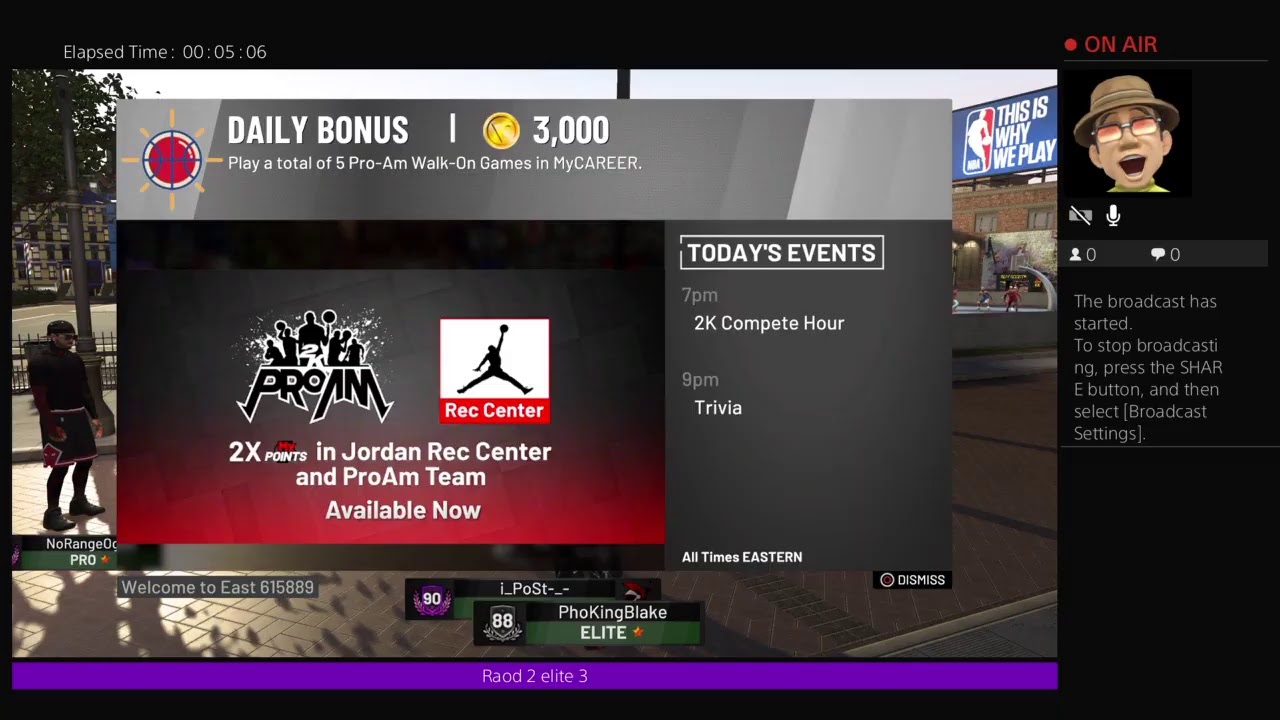The image depicts a section of a gaming website featuring a daily bonus notification. The notification reads “Daily Bonus: Play a total of five Pro-Am Walk-On games in MyCareer.” Adjacent to the daily bonus text is an icon resembling a sun, with yellow rays, a blue outline, a white rim, and a red inner circle. A gold circle displaying the number "3000" is prominently positioned at the top.

Beneath this, a black box with gray accents and a red bottom section is labeled "Pro-Am." Next to it, another box labeled "Rec Center" features a red bottom section and a white top. Within this box, there's an image of a basketball player mid-air, holding a ball. The caption reads “Two times points in Jordan Rec Center and Pro-Am team available now.”

The section also lists current events, stating “Today’s Events: 7 PM - 2K Compete Hour, 9 PM - Trivia (all times Eastern).” In the lower right corner, there is a “Dismiss” button.

This entire interface overlays a game-like background image. On the left side of this background, a character stands near a pole with shadows of leaves visible below. The right side features the slogan “This is why we play” over an NBA-themed image; everything rests atop a building. Below this is a white platform with a red character, and the text “Welcome to East 6 15 8 8 9.”

Moreover, a box indicating “90” is seen in purple beside the text "Pro King Blake Elite," with an “88” nearby and a purple bar running along the bottom. At the top of the interface, the phrase “On Air” is displayed in red, accompanied by an icon of a laughing character.